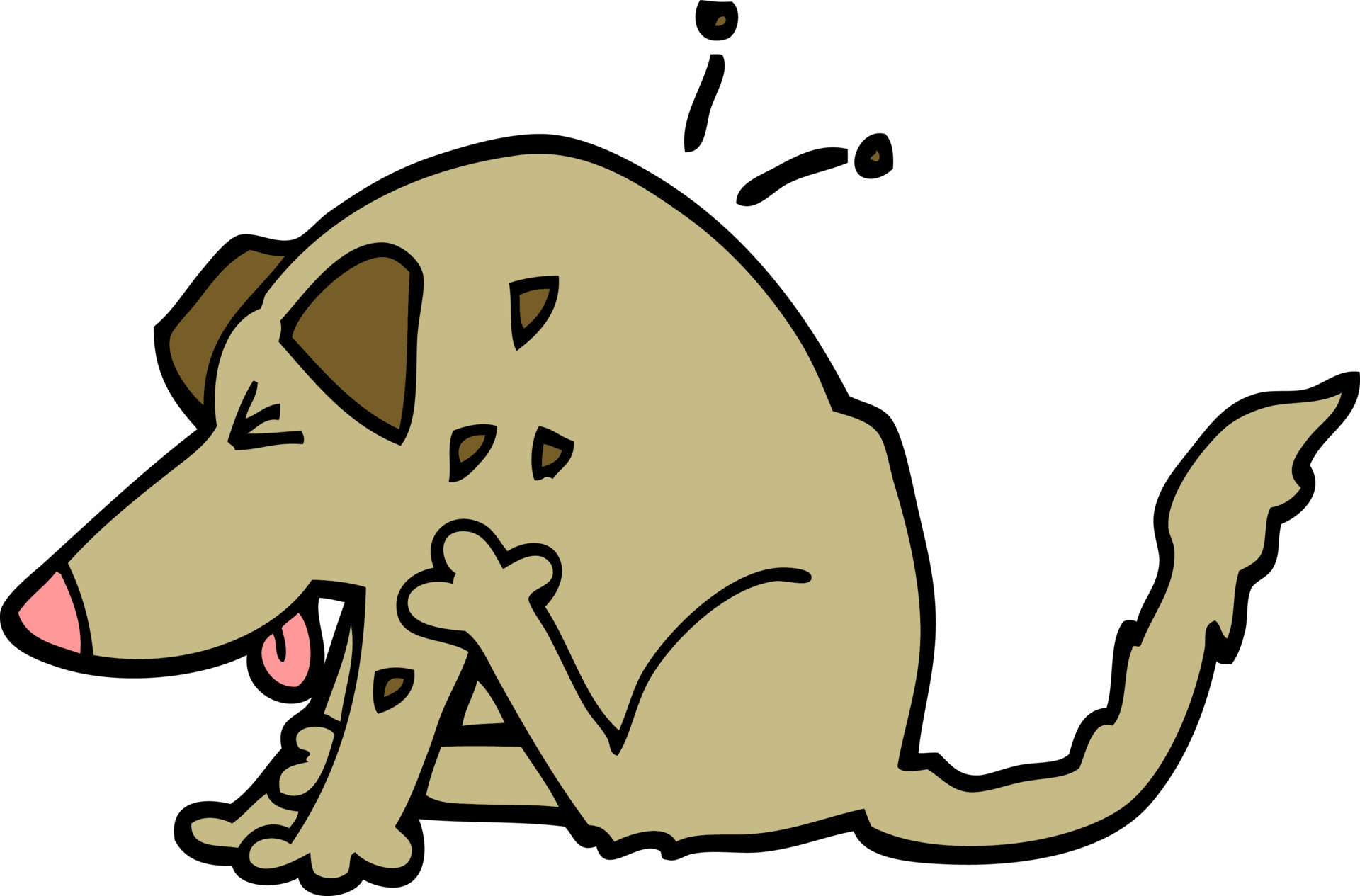This cartoon illustration depicts a light brown dog, almost khaki in color with a yellowish tint, actively scratching itself. The dog features darker brown ears and a couple of matching spots on its body. It has a pink nose and a pink tongue that hangs out from its open mouth. Its eyes are closed, indicated by three simple black lines for each eye. The dog is sitting to the left of the frame on its haunches with its two front paws planted firmly on the ground. Its right hind leg is extended through the front paws, while the left hind leg is raised and scratching its shoulder. Above its head, there are a couple of confused lines, possibly indicating motion or the dog's focused effort. Additionally, there are two black lines with dots at the ends coming off its back, suggesting the presence of fleas being dislodged as it scratches. The background is plain white, emphasizing the dog’s comical yet concentrated demeanor as it relieves its itch.